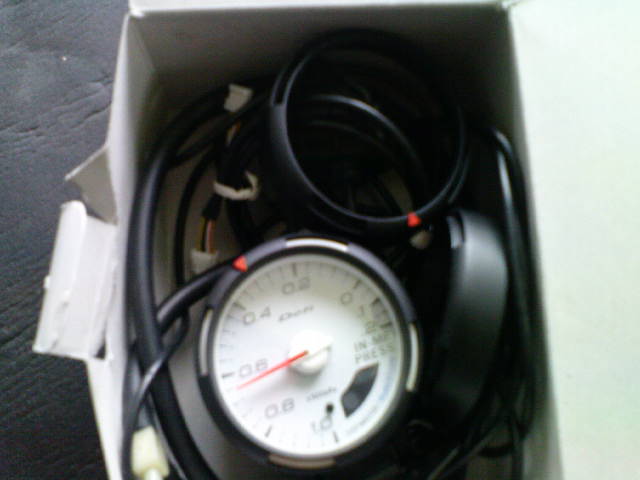The image depicts an old, white, rectangular box placed on a black surface, which is likely either a table or the floor. The box contains a tangle of randomly arranged black wires. Among the wires, there is a noticeable circular item resembling a bracelet with several openings and a red arrow at the bottom. To the right of this, another circular object is partially visible but not fully shown. Additionally, there is a third circular object that appears to be a covered circular watch, featuring a silver exterior.

Centered within the box, this circular item showcases a white background with numbers positioned around its edge. The visible markings include increments of 0.2, 0.4, 0.6, 0.8, and 1.0, marked in a consistent circular pattern. A red pointer is fixed at the 0.6 mark. Adjacent to these, there are additional numbered markings on the right side, though only the digits 0, 1, and 2 are somewhat discernible. The bottom right section of the box displays a small black bar. This detailed configuration suggests a mixture of electrical and mechanical components stored together.